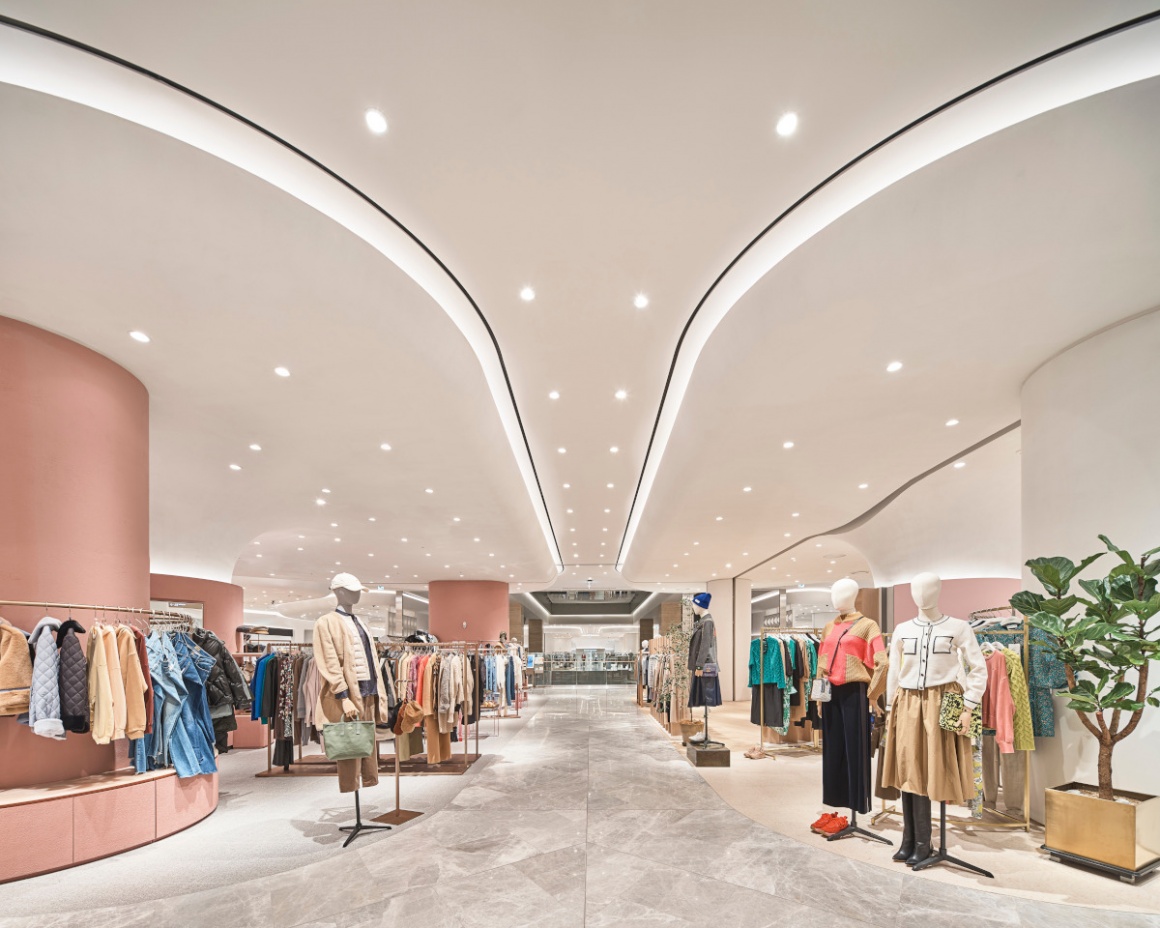This indoor photograph of a department store vividly showcases a spacious and well-lit women's section. The store features a mix of white and taupe or mauve-curved walls, complemented by marble flooring. Dominating the left side are rose gold-colored pillars situated at the front, middle, and back, adding an opulent touch. The white ceiling, adorned with multiple recessed light fixtures, brightly illuminates the space. 

The scene is bustling with a variety of mannequins, each dressed in distinct styles of women's clothing. On the left, a mannequin sports a jacket while holding a bag and a baseball cap, and surprisingly, a cone. To the right, three mannequins display different outfits: one wears a brown skirt paired with a white shirt featuring two pockets, another is dressed in a sweater and pants, and the third is clad in another unique ensemble. Additionally, a large potted green plant stands taller than the mannequins, adding a touch of nature to the sophisticated setting.

Racks of clothing, varying in style, color, and size, line both sides of a wide central path, inviting customers to explore. Overall, the department store exudes an inviting and luxurious ambiance, with meticulous attention to layout and design.